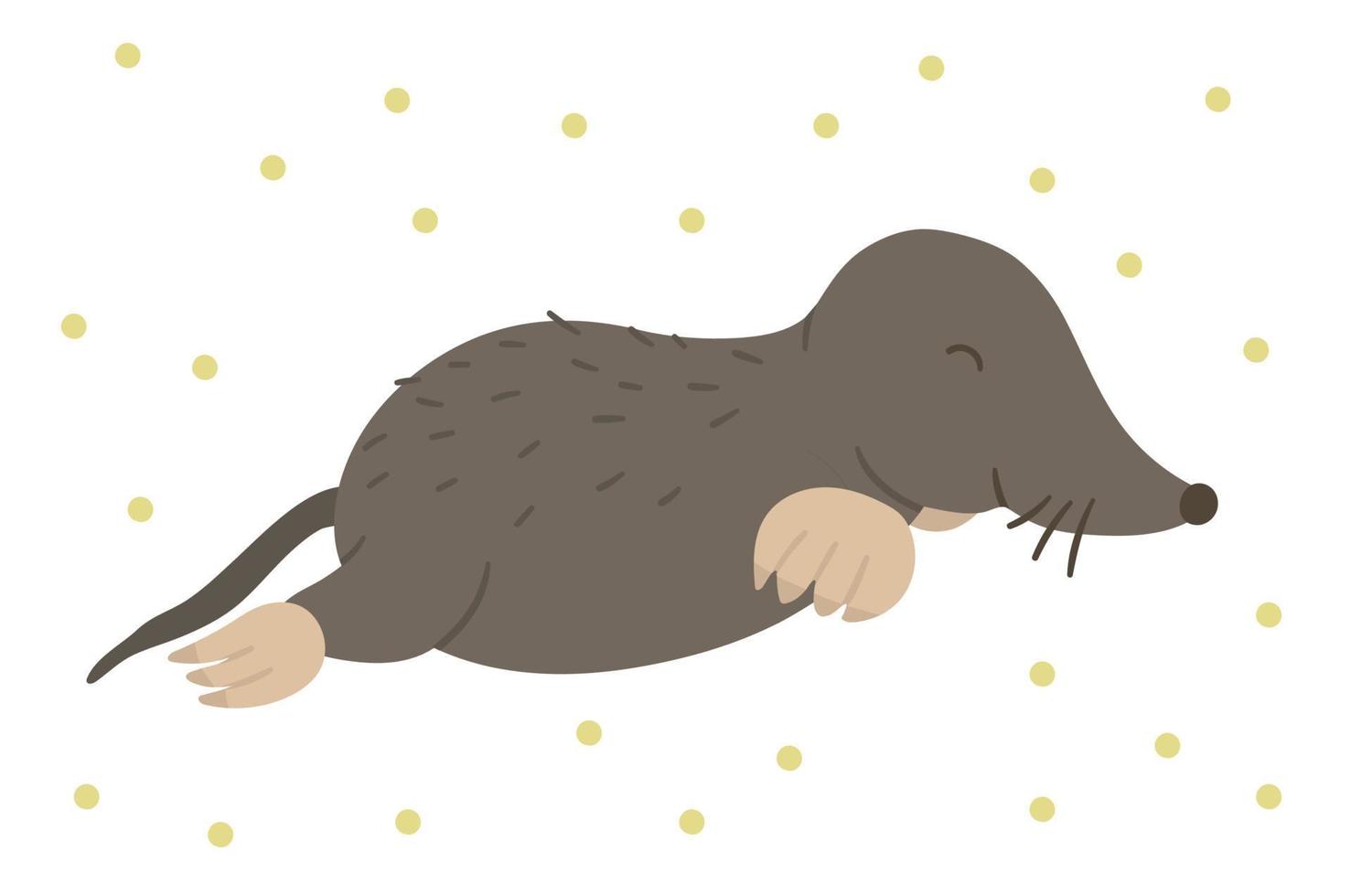This image illustrates a cartoon-style drawing of a mole set against a white background sprinkled with about 30 yellow dots. The mole, predominantly brown, is depicted in a resting position with its eyes closed, suggesting it's asleep. Its body is stretched out with all limbs extended, showcasing its human-like limbs with tan paws featuring four fingers on the front paws and three on the back. The mole's back displays patchiness, and it has a round, brown nose and long whiskers. Its head faces the right side of the image while a long, rat-like brown tail points to the left. The mole's anatomy includes a notably larger belly and distinct coloring with darker hues on the body and lighter shades on the paws.